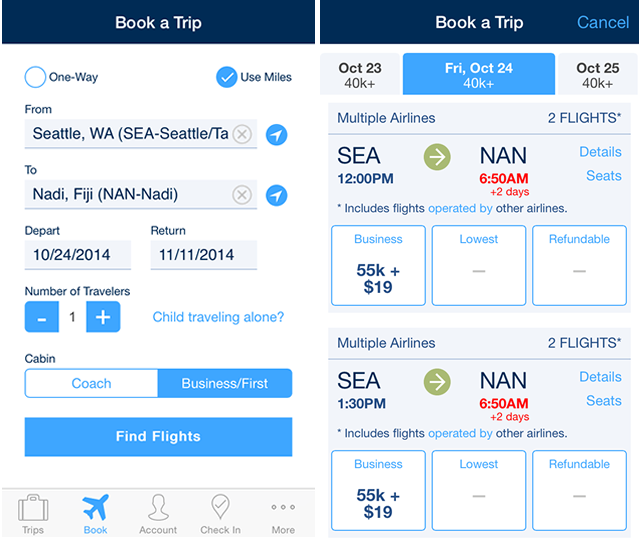This image contains two phone screenshots showcasing a trip planning interface. The top of each screenshot features a dark blue bar with the title "Book a Trip." On the right screenshot, a light blue "Cancel" option is visible.

The left screenshot displays options and fields for planning a trip. The "Use Miles" option is checked among the "One Way" and "Use Miles" choices. The trip details are filled in as follows:
- From: Seattle, Washington
- To: Nadi, Fiji
- Depart: October 24, 2014
- Return: November 11, 2014
- Number of travelers: One

There’s an inquiry about a child traveling alone that links to additional information. The "Cabin" section offers choices between "Coach" or "Business/First," with "Business/First" selected. Below, a blue button prompts to "Find Flights."

Lower on the screen, icons indicate different sections of the app:
- A gray suitcase labeled "Trips"
- A blue airplane labeled "Book"
- A head icon labeled "Account"
- A map pin labeled "Check-in"
- An ellipsis labeled "More"

The right screenshot shows the trip details for booking:
- Dates: Starting from October 23rd, highlighting Friday, October 24th
- Route: Seattle to Nadi (NAN)
- Business class pricing: 55,000 points plus $19
Alternate flight departing at 1:30 p.m. is listed with the same cost of 55,000 points plus $19, compared to an earlier time of 12:00 p.m.